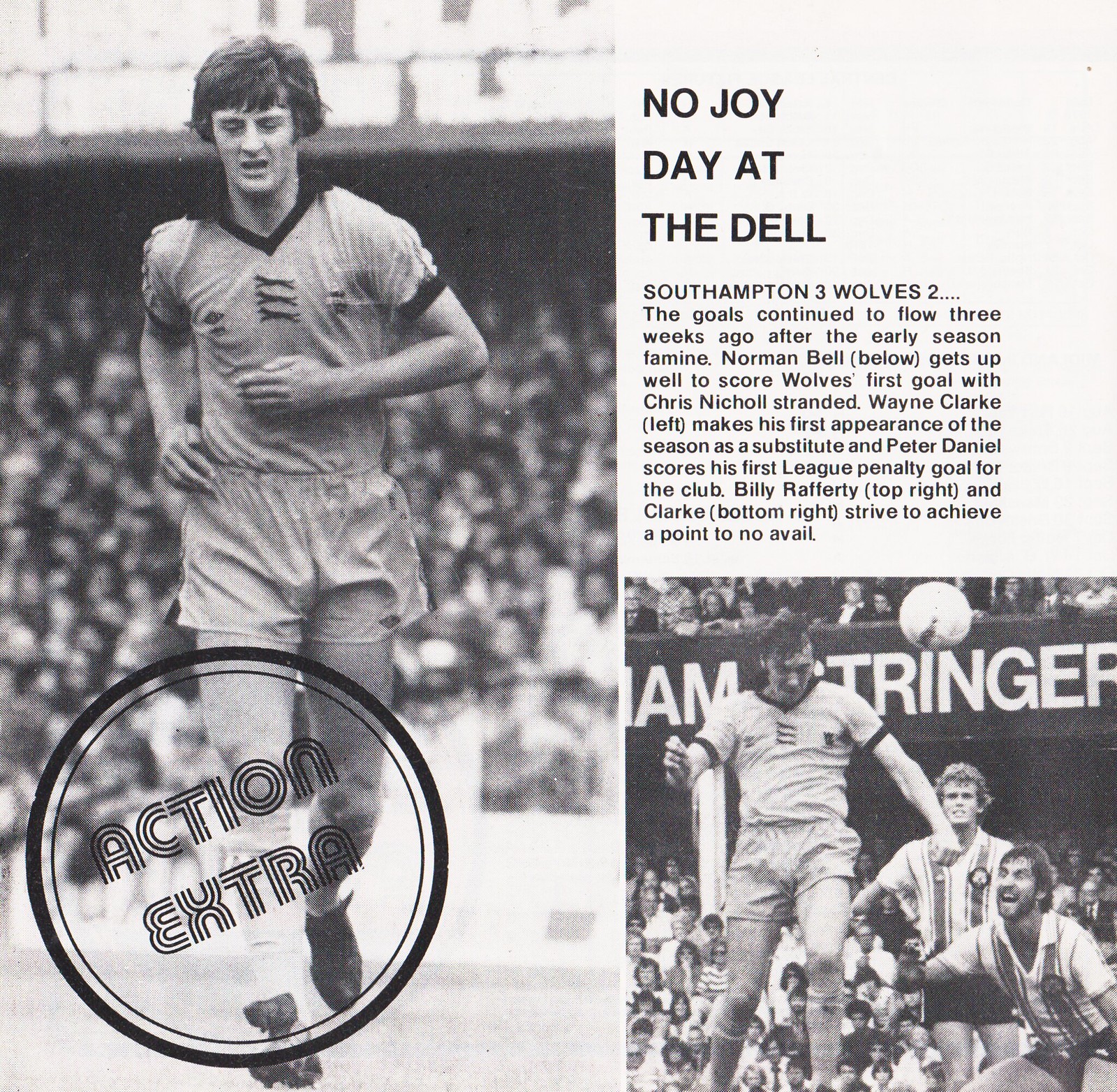This black and white newspaper or magazine article features dynamic images and text highlighting a soccer match between Southampton and Wolves. Dominating the left side of the image, a soccer player wearing a v-neck jersey is captured in motion, running with bent elbows and slightly bent knees, against a backdrop of a packed crowd in the bleachers. There's a circle overlay near his legs with the text "Action Extra." The headline at the top reads, "No Joy Day at the Dell, Southampton 3, Wolves 2," indicating an exciting game where the goals resumed after an early season lull. The detailed description continues to explain key moments: Norman Bell scoring Wolves' first goal with Chris Nichol stranded, Wayne Clark making his first season appearance as a substitute, and Peter Daniel netting his first league penalty goal. Additionally, Billy Rafferty and Wayne Clark, both pictured in the top and bottom right sections, strive for further points but are ultimately unsuccessful. The bottom right corner shows another part of the action, with a sign partially visible and players seemingly engaged in moments before hitting the ball, with one player in a v-neck shirt and others in striped and different patterned uniforms. The grayscale tones of the article and its well-positioned images give it a classic, archival quality, reinforcing it as a full-page spread dripping with nostalgia and historical sports significance.